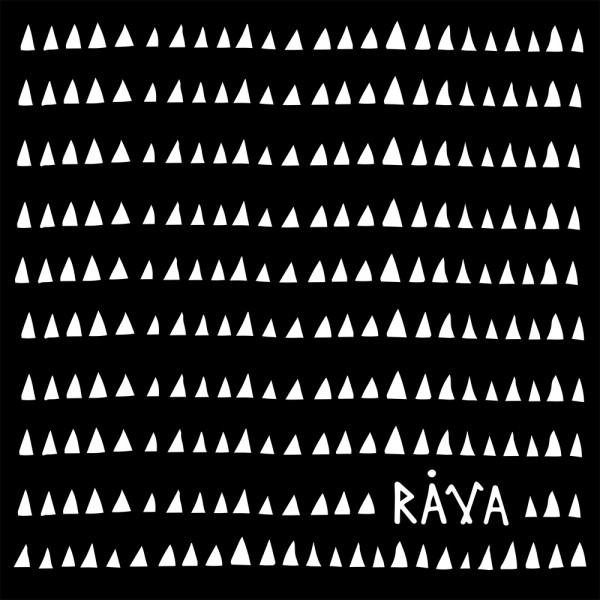The image features a black rectangular background, just slightly longer than it is wide, filled with numerous white, hand-drawn triangles arranged in horizontal rows. There are 10 distinct rows, each containing around 24 variably shaped triangles, with minor differences in size and shape adding a hand-drawn feel. The rows of triangles stretch evenly from left to right, creating a repetitive yet varied pattern. In the second to last row, positioned toward the bottom right, the white capital letters R-A-V-A are prominently displayed. The text interrupts the row and stands out due to its larger size compared to the surrounding triangles. The 'A' in 'Rava' has a dot above it, and the 'V' is stylized to look like a pair of golf clubs, adding a unique design element to the otherwise consistent triangular pattern. The entire image is monochromatic, with no borders or other objects, giving it a minimalistic yet intricate appearance.